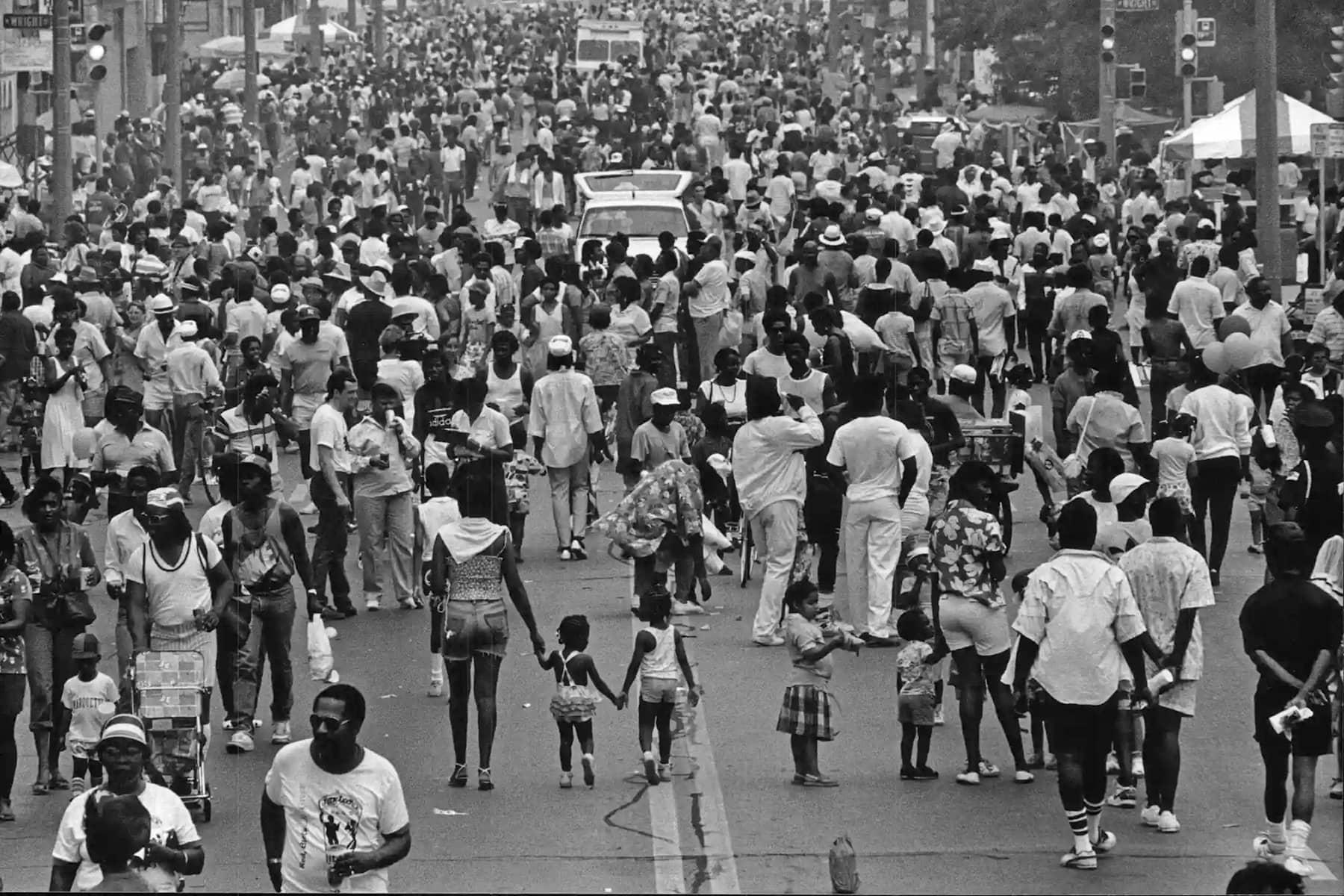This is a black-and-white photograph capturing a bustling scene on a wide, paved city road. A large crowd, including men, women, and children, fills the road, walking in both directions and covering a substantial portion of the street. Most people are dressed in white or grey clothes, and among them are individuals dressed in shorts and short-sleeved shirts, suggesting warm weather. Baby strollers and people holding hands are visible. A few cars are interspersed within the crowd, stopped due to the dense throng of people, hinting at a significant event, possibly a summer festival. On the sides of the road, traffic lights, signboards, power lines, and a glimpse of buildings are evident. Additionally, there's a visible tent top on the right-hand side and an umbrella that might be part of a stand. In the background, a fan can be seen.